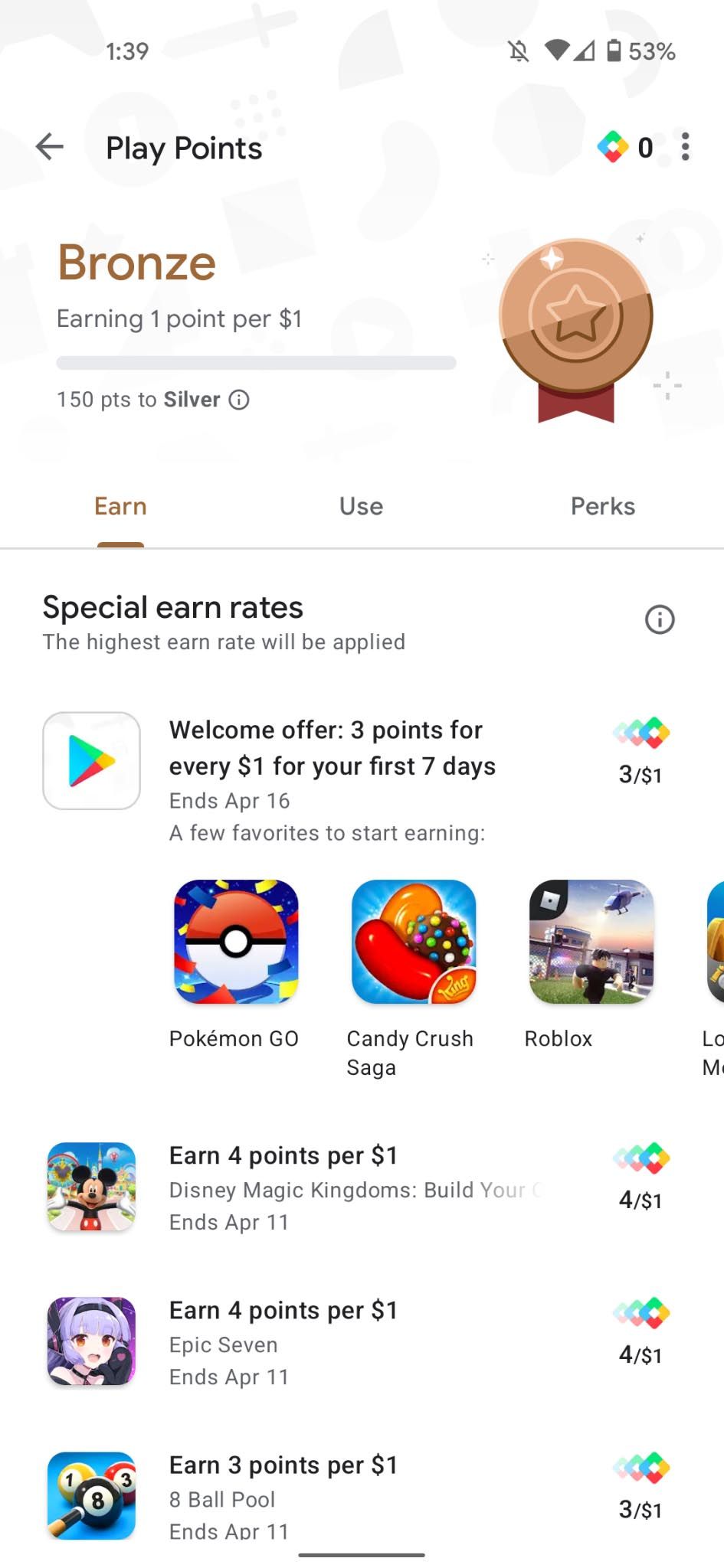A screenshot depicts a user's game reward screen, showcasing their progress within a play points system. At the top, the user has earned one point per dollar, achieving the Bronze tier, illustrated by a bronze medal featuring a star encircled by two concentric rings. The medal is adorned with a reddish ribbon. Below this, there's a notification stating "150 points until you reach Silver," accompanied by an information icon enclosed in a gray circle.

Further down, headings such as "Earn," "Use," and "Perks" can be seen, highlighting different aspects of the reward system. The section below specifies ways to earn more points, including "special earn rates" where the highest rate will be automatically applied. A prominent button for the Play Store explains a "welcome offer" of earning three points per dollar spent during the first seven days, ending on April 16th.

Highlighted games under "A few favorites to start earning" include popular titles like Pokémon Go, Candy Crush Saga, and Roblox. The detailed earning rates are prominently displayed: "Earn 4 points per $1" and "Earn 3 points per $1," encouraging users to engage more with these games to maximize their rewards.